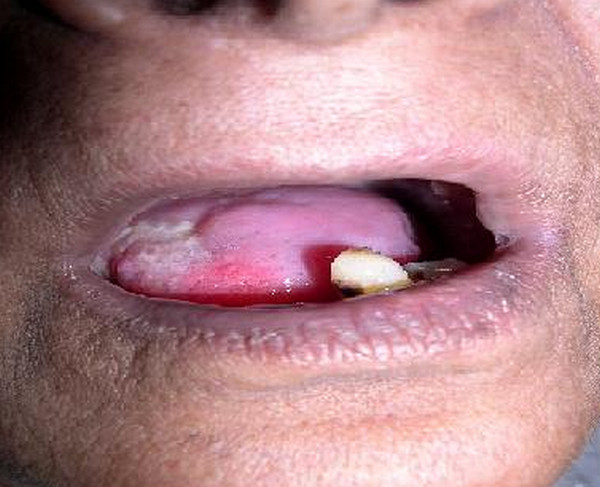The image depicts an extreme close-up of an elderly African-American man's mouth, slightly open to reveal significant dental and oral health issues. His chapped lips are a faded maroon color, and the close-up frame also captures a bit of his tan skin under the nose and just past the chin. Inside the mouth, a single, crooked, and rotten tooth juts awkwardly from the lower right side, almost lying flat. His tongue appears pink but is marred by white growths and red sores, with some blood possibly visible near the front. The stark detail suggests the man is suffering from severe periodontal disease, characterized by the loss of most of his teeth.